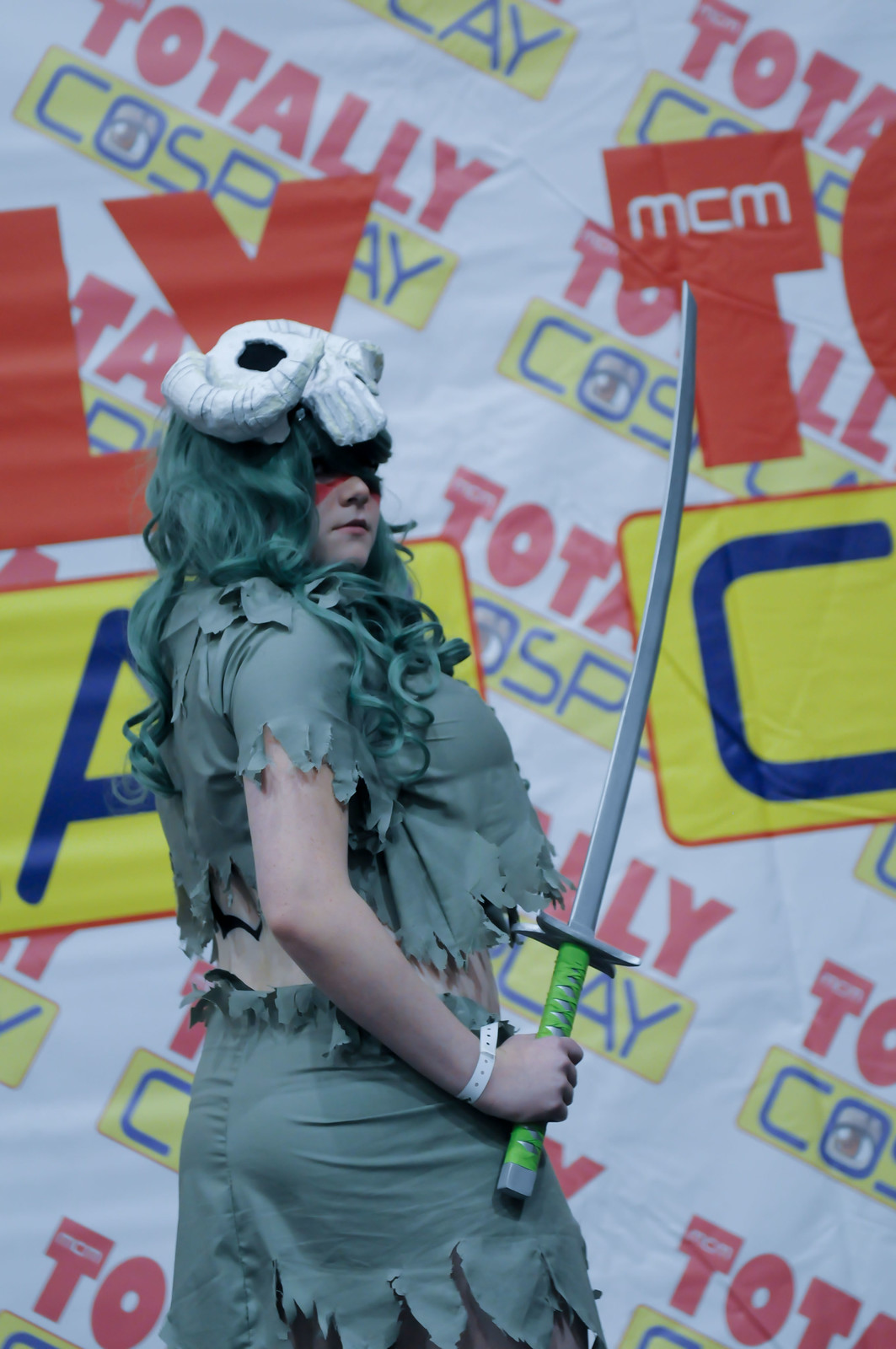The image depicts a cosplayer standing in front of a banner at a cosplay convention. The individual, whose gender is ambiguous, is wearing a ragged, greyish top and skirt, giving off an intentionally distressed look. They have a grey-green wig adorned with what appears to be a paper mache ram skull with protruding horns. Partially turned with her back to the camera, the cosplayer holds a katana with a green, taped hilt in their right hand. Her eyes are obscured by the wig, adding to the dramatic appearance. Behind her, the prominent backdrop reads "Totally Cosplay," with "Totally" in red and "Cosplay" in blue font on a yellow background. The letter "O" in "Cosplay" features a brown anime-style eye.